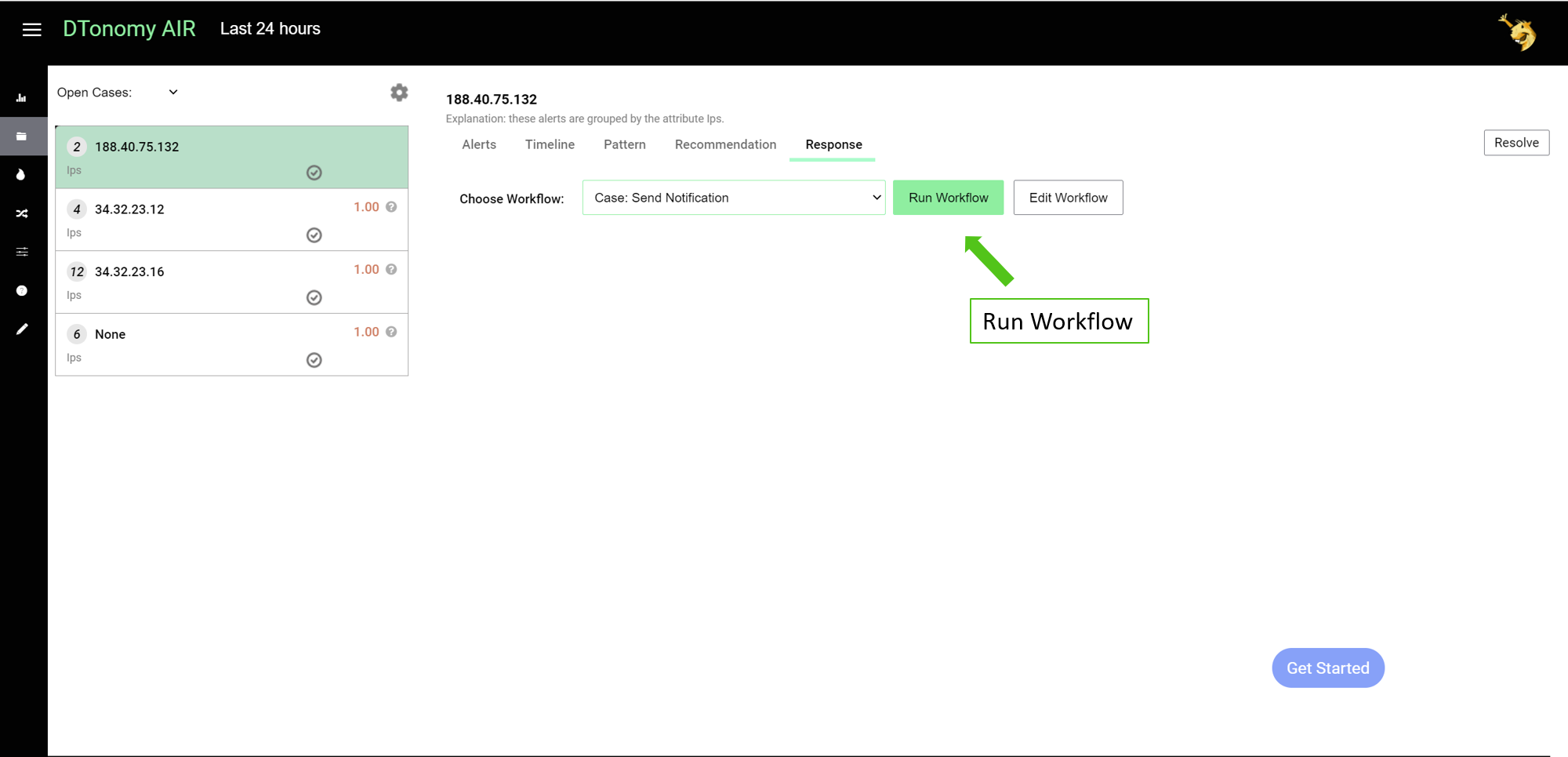In the screenshot, there is a distinctive black header and a black navigation bar situated on the left side. At the top, prominently displayed in green text, is the phrase “D Tono My Air,” followed by “last 24 hours” in light gray text. An icon resembling a cartoon-like woodchuck's face, illustrated in brown, occupies the upper right corner of the header.

Against the white background of the main screen area, bold numbers “188.40.75.132” are prominently featured. Directly beneath these numbers, light gray text provides an explanation, stating, "These alerts are grouped by the attribute LPS."

Below the explanation, a horizontal menu spans from left to right, listing the following options: "Alerts," "Timeline," "Pattern," "Recommendation," and the underlined "Response." Situated further below is a green highlighted button labeled "Run Workflow." Directly beneath this button, a large green arrow points upward, drawing attention to the button.